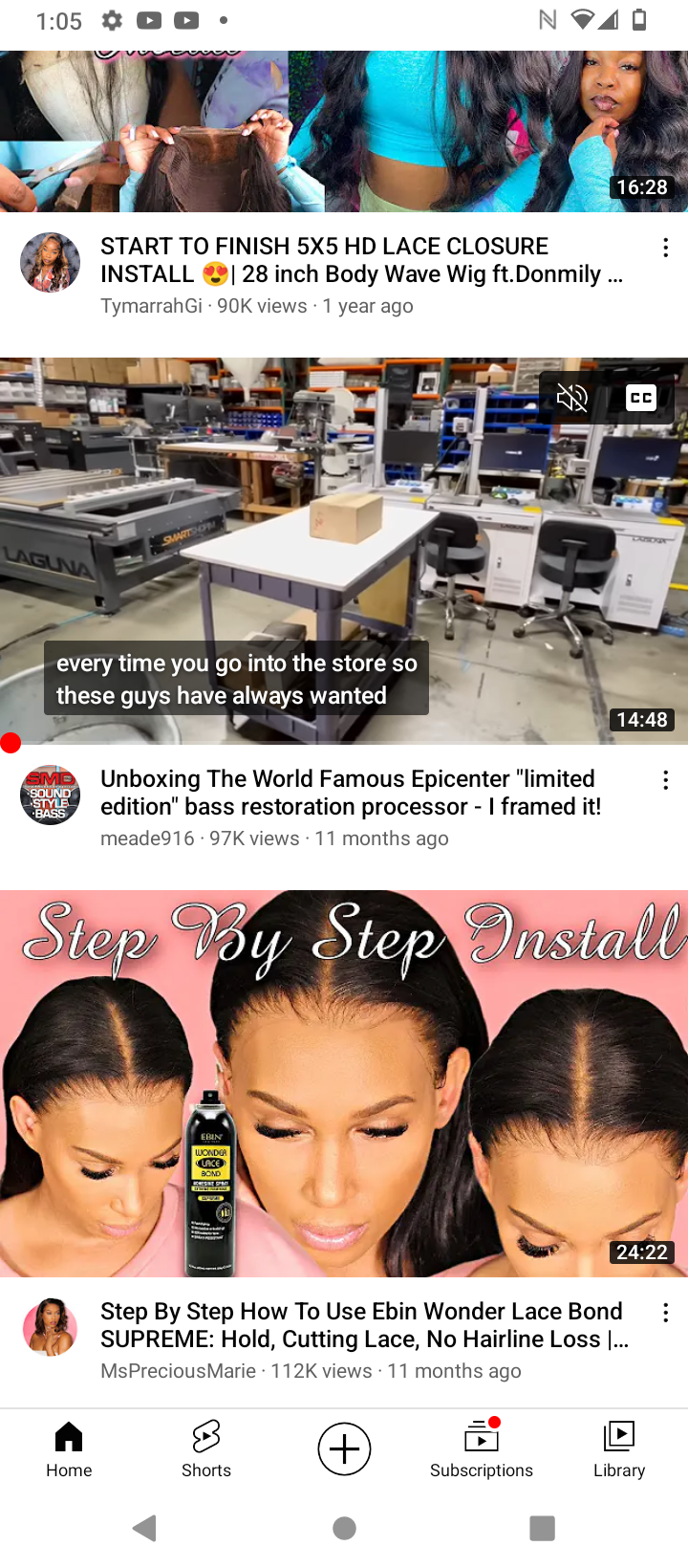The image depicts a screenshot of a mobile device displaying a web page, likely a video-sharing platform such as YouTube. At the very top, there is the status bar indicating the current time, battery level, and signal strength along with other icons. Below this, a thin horizontal strip features several thumbnail images, predominantly of women, suggesting they could be video thumbnails or profile pictures. Further down, a round profile picture is positioned beside a line of black text. 

Continuing down, a larger, thicker rectangular section showcases a complex image featuring various tables and objects, hinting that it might be an instructional or review video, though its exact content is unclear. Another round profile picture appears with another text block to its right. 

Following that, a rectangular banner reads "Step-by-Step Install" in white text, accompanied by three sequential images of a woman's head showcasing a hair installation process. Yet another round profile picture is paired with black text. At the bottom of the screen, navigation icons for home and additional features such as subscription, library, and search are visible alongside a gray left arrow and gray box indicator, further confirming the mobile interface. The video content seems centered around hair products and installation tutorials, alongside other potentially unrelated videos.